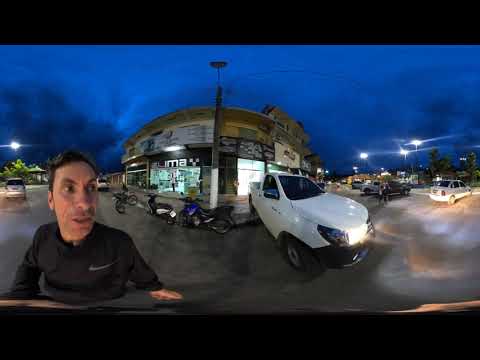In the image, a skewed photograph captures a street corner scene, possibly depicting a restaurant or store. A small white pickup truck with headlights on is backed up against the curb, partially on the sidewalk. The setting is outdoor with a deep blue sky, indicating it's either nighttime or the sun is rising or setting. Several vehicles are present: a white sedan, a black sedan, and a few motorcycles parked outside the building, which is centrally located in the frame. Streetlights are illuminated, contributing to the image's dim atmosphere. In the foreground, a man dressed in a long-sleeve black t-shirt stands near the bottom left corner of the image, facing towards the camera but not directly looking at it. The photograph also features a streetlight on the left side and a sign on the building that reads "IMAY," suggesting it is in a parking lot with additional cars surrounding it. The sky, painted with shades of dark blue and black clouds, enhances the late evening or early morning feel of the scene.